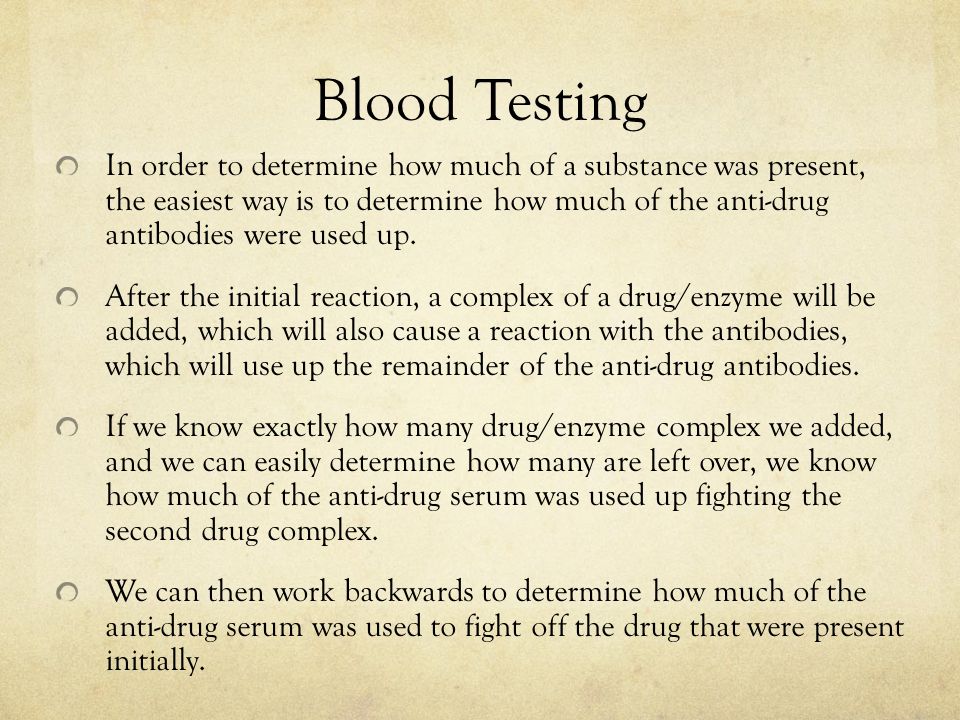The image features a PowerPoint slide with a tan background and dark-colored text, taking up the entirety of the image. The title, "Blood Testing," is prominently displayed at the top in bold. Below the title, four bullet points outline the process of determining how much of a substance is present in a blood sample by analyzing anti-drug antibodies:

1. To determine the amount of a substance present, the easiest method is to measure how much of the anti-drug antibodies were used up.
2. After the initial reaction, an enzyme-drug complex is added, which also reacts with the antibodies, consuming the remaining anti-drug antibodies.
3. Knowing the exact amount of enzyme-drug complex added and how much remains, we can calculate how much anti-drug serum was used up fighting the second complex.
4. By working backwards from this data, we can determine the amount of anti-drug serum used to combat the initial drug present.

This detailed caption provides a clear and comprehensive description of the blood testing process, as presented in the image.